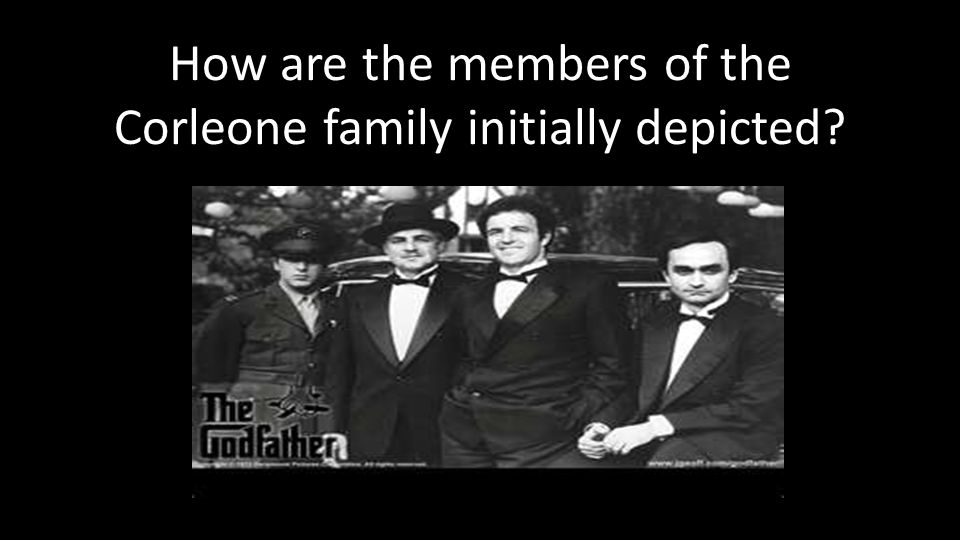The black and white photograph depicts a promotional image from the movie "The Godfather," featuring four key characters from the Corleone family. At the top of the image, a caption in bold white letters asks, "How are the members of the Corleone family initially depicted?" In the lower-left corner, the iconic logo of "The Godfather" is displayed. The background is completely black, framing the subjects prominently. 

From left to right, the characters are positioned in front of an old car, which hints at the 1940s setting of the movie. On the far left stands Al Pacino's character, Michael Corleone, dressed in a military uniform complete with a hat, signifying his time in the army. Next to him is Marlon Brando as Don Vito Corleone, wearing a tall hat, a black suit, a white shirt, and a black bow tie. To his right is James Caan, portraying Sonny Corleone, also dressed in a black suit, white shirt, and black bow tie, but without a hat. On the far right stands John Cazale's character, Fredo Corleone, similarly attired in a black suit, white shirt, and black bow tie, without a hat. The men appear to be leaning against the car, with all of them smiling except Sonny and Fredo. The detailed setting and attire highlight the film's period and the characters' personalities and roles within the family.